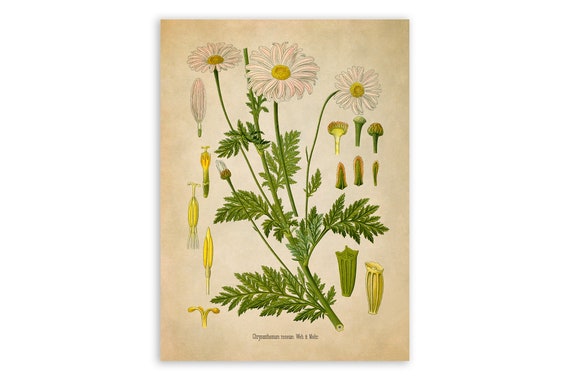This poster displays a detailed, old scientific illustration of chrysanthemums, showcasing their development stages from bud to full bloom. The centered chrysanthemum plants are depicted with green stems and leaves, resembling parsley in their delicate branching. The flowers have white petals with vibrant yellow centers, and some buds show hints of yellow as they start to blossom. To the left and right of the central images, smaller illustrations break down various parts of the chrysanthemum, albeit without labels. The beige background of the poster, along with the small text at the bottom possibly indicating the scientific name, emphasizes its vintage, educational nature. Overall, the poster intricately captures the growth and anatomy of chrysanthemums from initial budding to fully blossomed flowers.